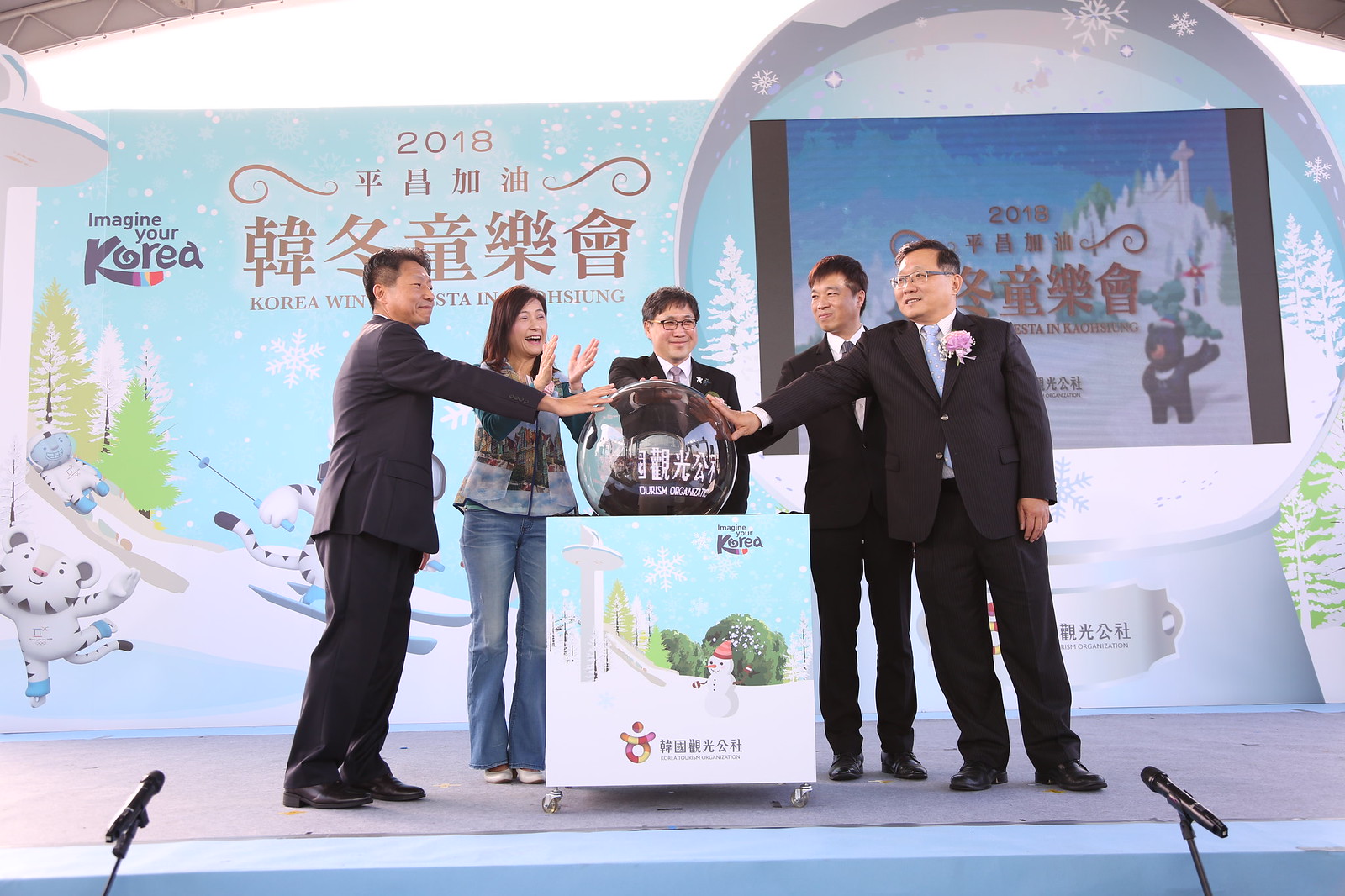In the image, five people are gathered on a stage, all engaged in an activity centered around a large, clear sphere, possibly made of glass or crystal, which has Korean writing on it. Positioned prominently in front of a banner that reads "2018" along with Korean symbols, the scene suggests a celebration or ceremonial event in Korea, potentially related to a winter festival or the Winter Olympics. Four men, all wearing black suits with flowers in their lapels, have their hands placed on the sphere, while a woman dressed in blue jeans and a blue patterned shirt claps and laughs. The background displays a snowy mountain with cartoony characters skiing or sledding down, reinforcing the winter theme. Microphones are set up at the bottom left and right sides of the stage, although no one appears to be speaking, making it clear they are posing for the photo. The atmosphere is festive and coordinated, possibly showcasing an important cultural or celebratory moment.